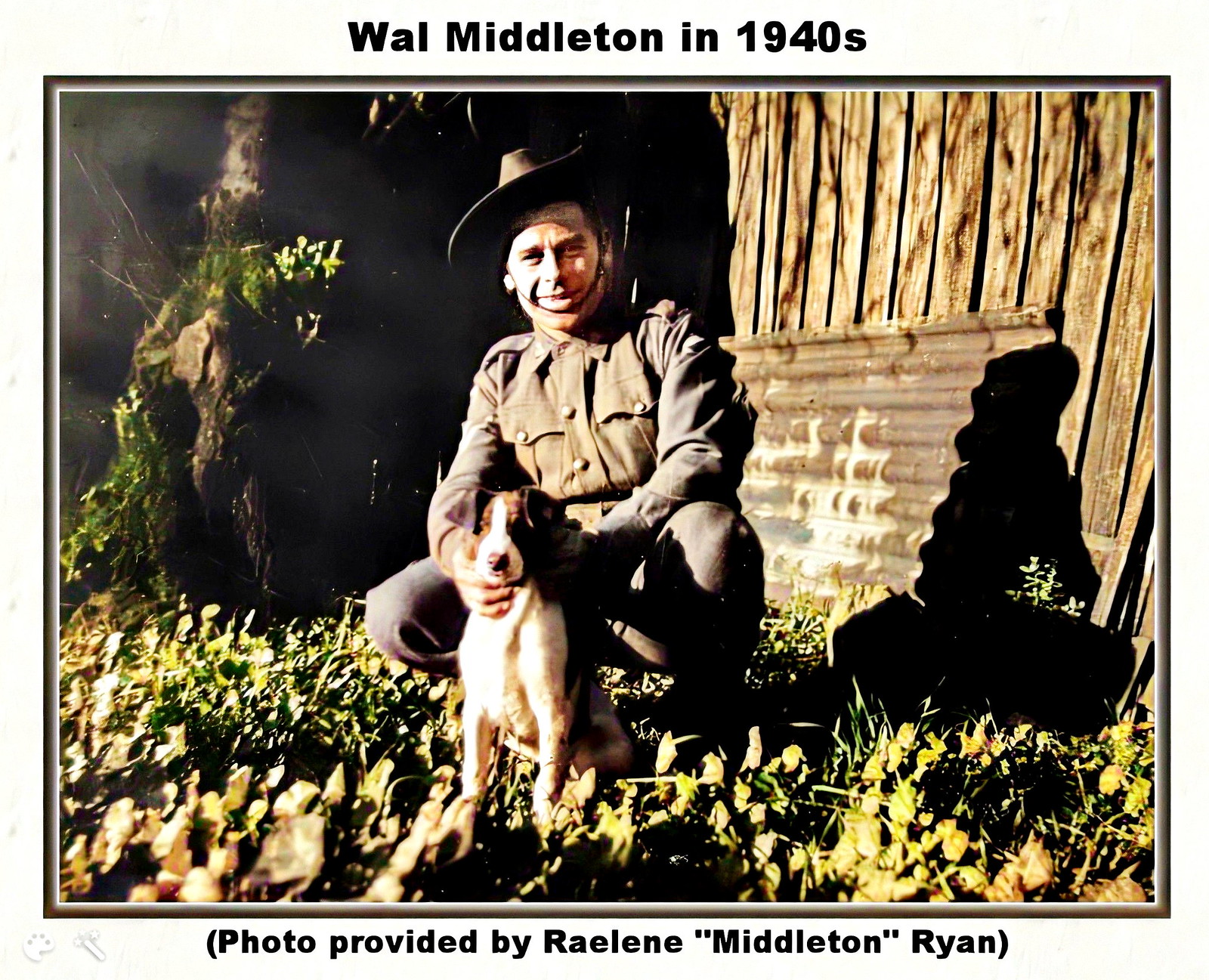The photograph, framed by a white and thin darker brown inner border, captures Wall Middleton in the 1940s, as indicated by black text on the upper white border. The lower border notes that the photo is provided by Raleen Middleton Ryan. In the center, a soldier, Wall Middleton, is squatting on a grassy area with some visible weeds. He wears a slightly curved-brim hat with a chin strap around his lower lip and a tan military uniform adorned with brass buttons. Middleton, a white man, smiles directly at the camera while holding his medium-sized brown and white dog with drooping ears, ensuring it looks forward. The background reveals a part of a tree and a wooden wall, adding depth to the scene.